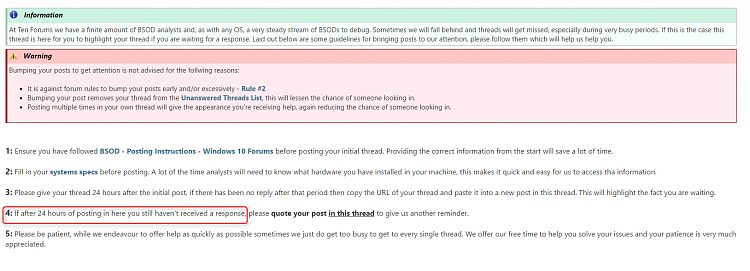The image displays comprehensive information and warnings pertinent to a forum. At the top, a long rectangular section with a green header labelled "Information" contains the following message:

"At 10 forums, we have a finite amount of BSOD analysis, and as with any OS, a very steady stream of BSODs to debug. Sometimes we will fall behind and threads will get missed, especially during very busy periods. If this is the case, this thread is here for you to highlight your thread if you are waiting for a response. Laid out below are some guidelines for bringing posts to our attention. Please follow them, which will help us help you."

Beneath this, there's a reddish rectangle featuring a red header titled "Warning: Bumping Your Post" with the text:

"Bumping your post to get attention is not advised for the following reasons. It is against forum rules to bump your posts early and/or exclusively. Rule number two, bumping your post removes your thread from the unanswered threads list. This will lessen the chance of someone looking in. Posting multiple times in your own thread will give the appearance you are receiving help, again reducing the chance of someone looking in."

Following this warning, a list of five steps is provided for users to follow. The fourth step is overlaid with a red rectangle for emphasis, stating:

"If after 24 hours of posting in here, you still haven't received a response, please quote your post in this thread to give us another reminder."